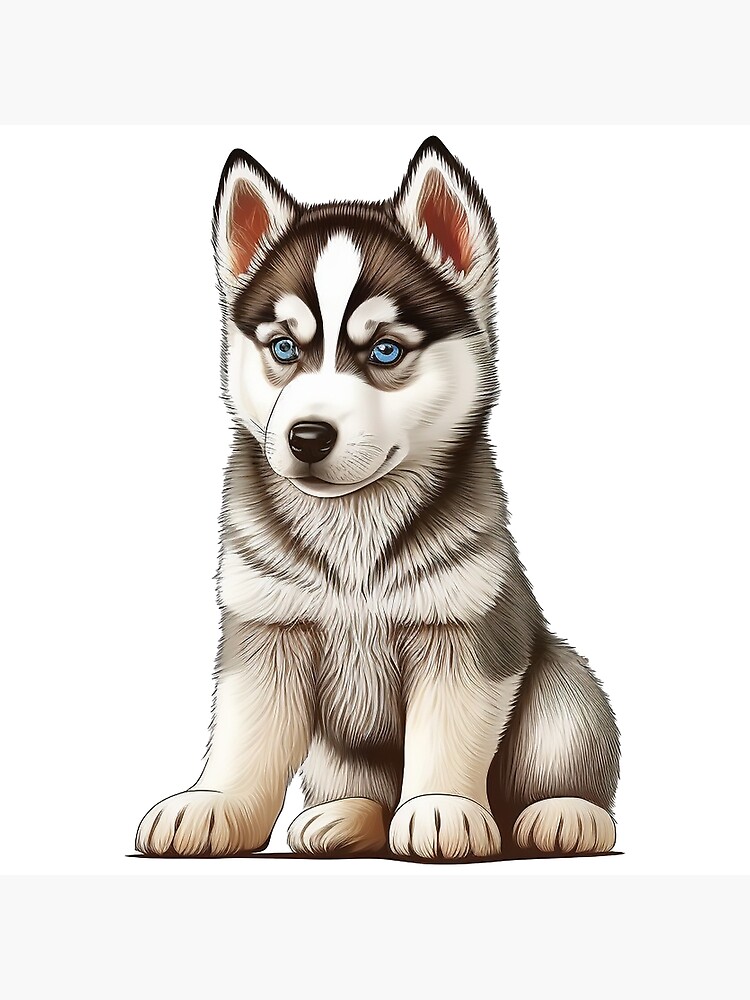This artwork depicts an endearing husky puppy rendered in a meticulous etching style, dominated by cream and gray tones. The pup, characterized by its striking sharp blue eyes, sits on its haunches with four white paws. The fur transitions from a darker gray to a whiter chest, adorned with subtle gray stripes. Its face showcases distinctive husky markings with a black raccoon-like mask around the eyes, complemented by expressive white eyebrows and a white line running up from its shiny button nose, which is brown rather than black. The puppy's ears are charmingly alert, standing upright with pinkish-red interiors and a black outline. Additionally, delicate whiskers sprout from its nose. Set against a plain white background, this drawing vividly captures the puppy's alert and friendly expression, making it irresistibly adorable.